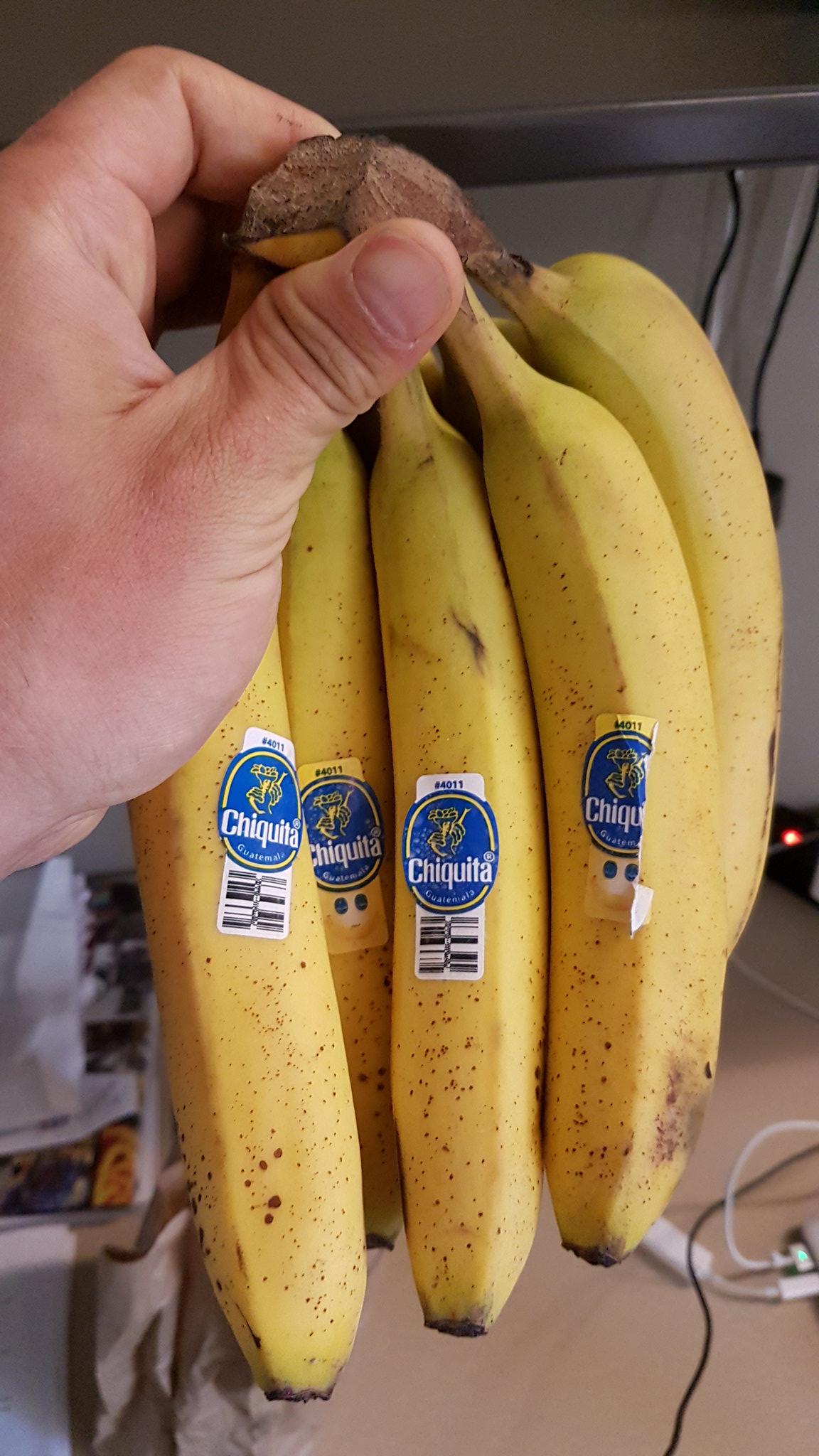A photograph captures a bunch of Chiquita bananas held vertically by a white man's left hand, which has clear nail polish-free nails. The bananas, numbering approximately eight with four in the front row each bearing the blue Chiquita sticker, are mostly yellow with a slight lime-green tinge at the top stem and starting to speckle brown at the bottom. One of the stickers on the top right banana is peeling off. The background reveals various cords, a charger port, a black monitor or TV, and a small table with printed pictures on its frame and a white paper bag.